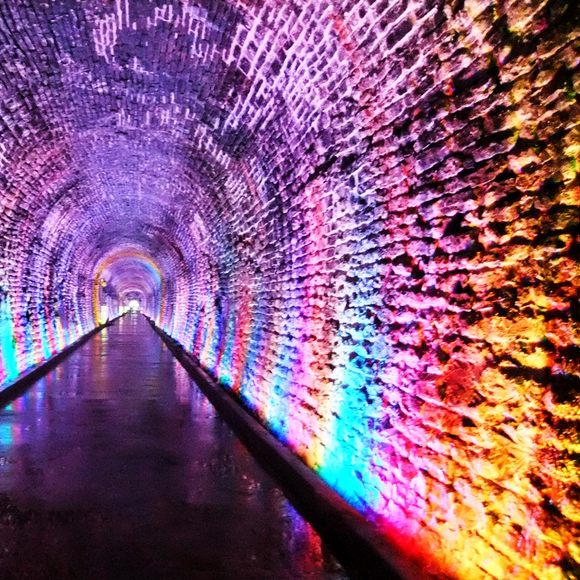The image depicts an eerie, surreal tunnel that gives the impression of a disorienting, dreamlike experience. The walls, made of very thin and small bricks, create an unusual and unsettling texture that almost appears to be alive due to their granulated look. The tunnel structure arches overhead, with thin, brick-like walls that curve inwards, creating a feeling of confinement. LED lights are strategically placed along the edges of a concrete or stone pathway, casting vibrant, rainbow-colored hues—yellows, oranges, pinks, purples, and blues—that illuminate the entire tunnel. These colors cycle in a repeating pattern, contributing to a psychedelic ambiance, reminiscent of an acid trip. The pathway features occasional divots, enhancing the strange and uneven feeling underfoot. Despite its odd appearance, the tunnel serves a functional purpose, likely providing passage within an urban development area, and is brightly lit to ensure visibility and safety at night. The black barriers on either side of the walkway flank the lit-up walls, leading the observer to an enigmatic journey through a kaleidoscopic passage.